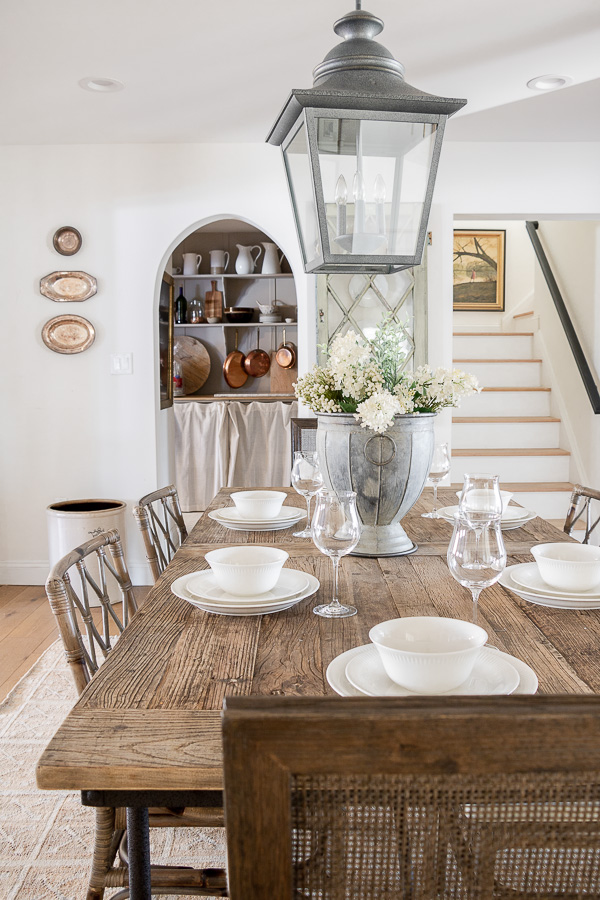The photograph captures the interior of a pristine dining room, which may also serve as a kitchen space. The room's farmhouse style is underscored by its white walls and ceiling, as well as a white staircase partially visible on the right, featuring a black rail and a painting in muted golden and tan tones. The focal point is a wooden dining table surrounded by six wicker chairs, each place setting carefully arranged with a stack comprising a white dinner plate, a salad plate, and a bowl, complemented by clear wine glasses. At the center of the table is a metal bucket filled with dried, white flowers serving as the centerpiece. To the left of the table, an antique display nook houses assorted pots, pans, pitchers, and glass jars not in everyday use, accompanied by three decorative silver plates—one round and two oblong—pinned to the wall. Above the table hangs a large gray light fixture, illuminating the room's thoughtful and clean aesthetic.